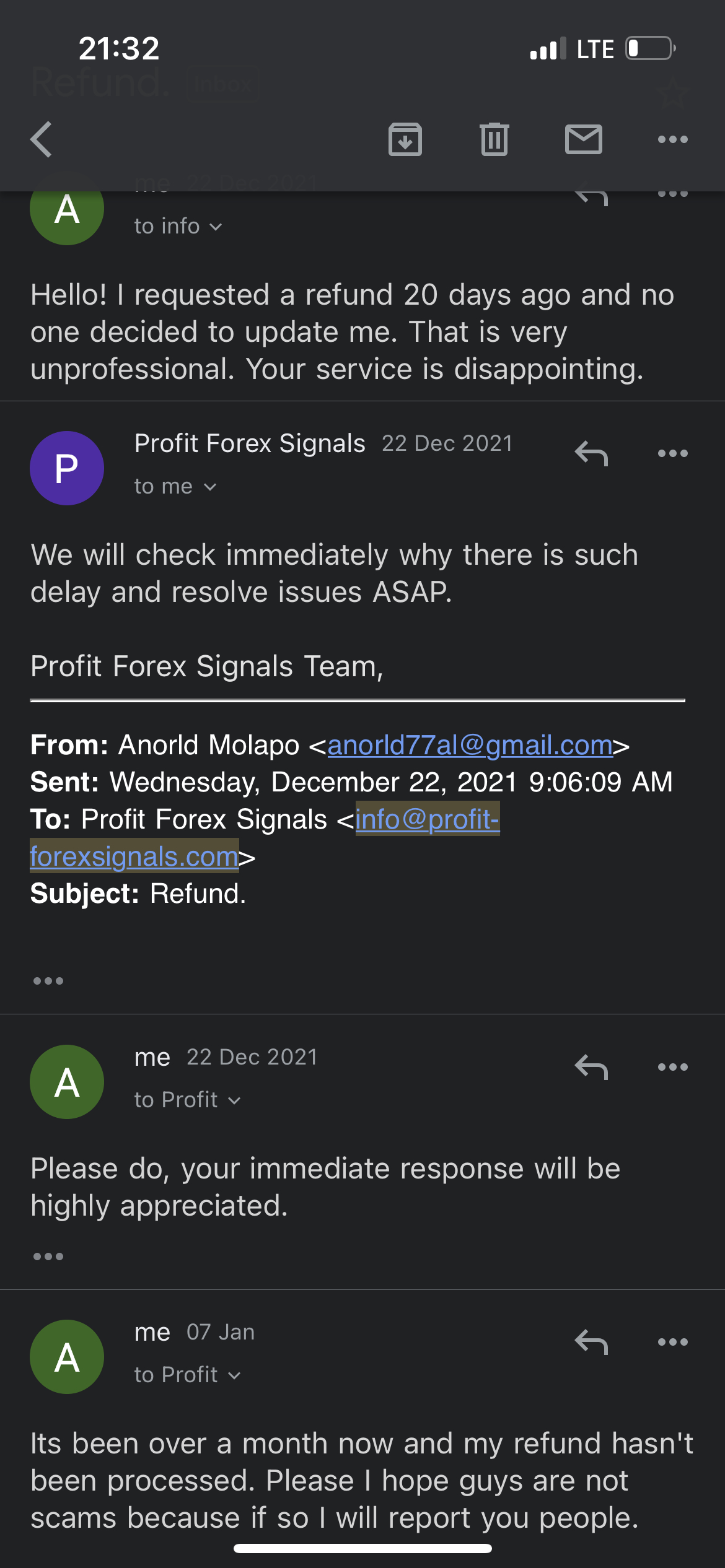Screenshot of a smartphone displaying a messaging app conversation. The top of the screen shows standard phone icons: a black area on the upper left shows the time as "21:32", the right side indicates almost full cell signal strength with LTE, and about a quarter left of battery life. Below, on the left, there is a back arrow in gray, and on the right are three vertical dots. 

The messaging conversation begins with a green circle featuring an "A" indicating the user: "Hello, I requested a refund 20 days ago and no one has updated me. This is very unprofessional. Your service is disappointing." The reply, from a "P" (possibly "Profit"), dated December 22, 2021, reads: "We will check immediately why there is such a delay and who is handling it. ASAP, Profit." 

Following this, the user sends another message: "Please, your immediate response would be highly appreciated." Finally, on January 7th, the user states: "It's been over a month. I hope you guys are not a scam because I will have to report you."

Commentary added at the end of the conversation expresses frustration and suspicion, suggesting that the company seems scam-like due to the prolonged refund process. The conversation ends with the decision to move on from this service.